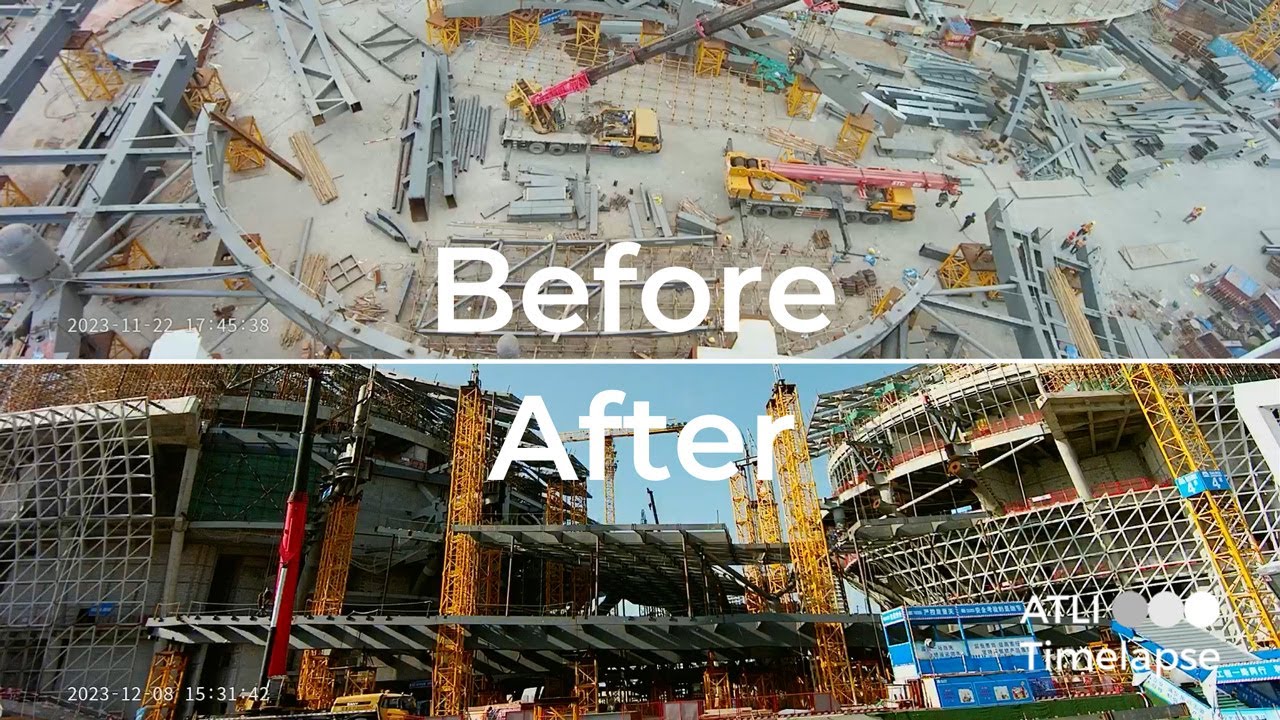The image features a split view of a stadium construction site, showcasing a "before" and "after" scenario. The top half, labeled "before" in bold white lettering, presents an aerial view of the initial construction stages. The site is cluttered with various metal pieces and fixtures, and you can see two red trucks with silver beds hauling materials. One of these trucks has a long red crane. The ground is bare and dusty, emphasizing the chaotic early phases of construction.

In contrast, the bottom half of the image, labeled "after," displays a side view of the now-completed stadium. The structure is fully erected, with all the metal components seamlessly integrated into the building’s framework. The lower right corner of this image segment contains the text "ATL-1" with "time lapse" underneath it, along with three circles in varying shades of gray and white. Additionally, there is a date and timestamp, "2023-12-08" and "1531-42," in small white lettering in the bottom left corner, marking the time frame of the transformation.